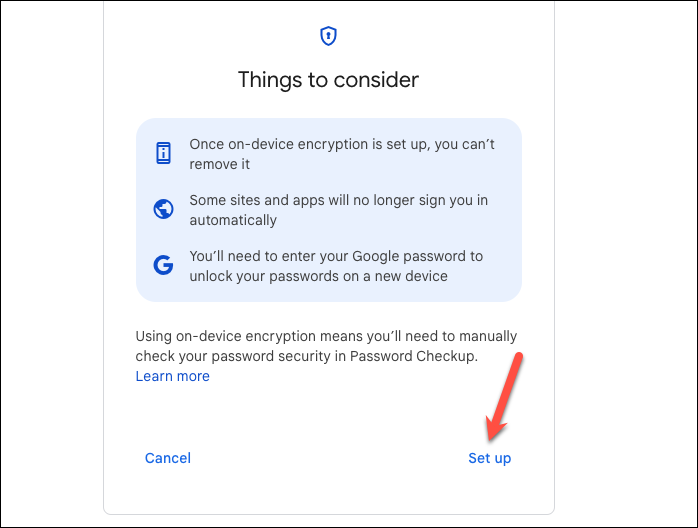The image features a black border surrounding a white central area. About a quarter of the way in from both the left and right sides, there's a gray horizontal bar. In the center of this gray bar is a shield icon with a vintage keyhole design against a blue background. 

At the top of the main white section, there is black text that reads, "Things to consider." Below, a blue column on the left side displays a sequence of icons: a phone, a globe, and the Google 'G.' To the right of each icon is corresponding black text:

1. "Once on-device encryption is set up, you can't remove it."
2. "Some sites and apps will no longer sign in automatically."
3. "You'll need to enter your Google password to unlock your passwords on a new device."

Further down on the white background, it states, "Using on-device encryption means you'll need to manually check your password security and password checkup." 

At the bottom left, there's a link labeled "Learn more." Additionally, on the bottom left-hand side, there's a "Cancel" button, both in blue. On the bottom right-hand side, there's a "Set up" button, highlighted by a red arrow pointing down at it.

This detailed overview captures all elements present in the image.